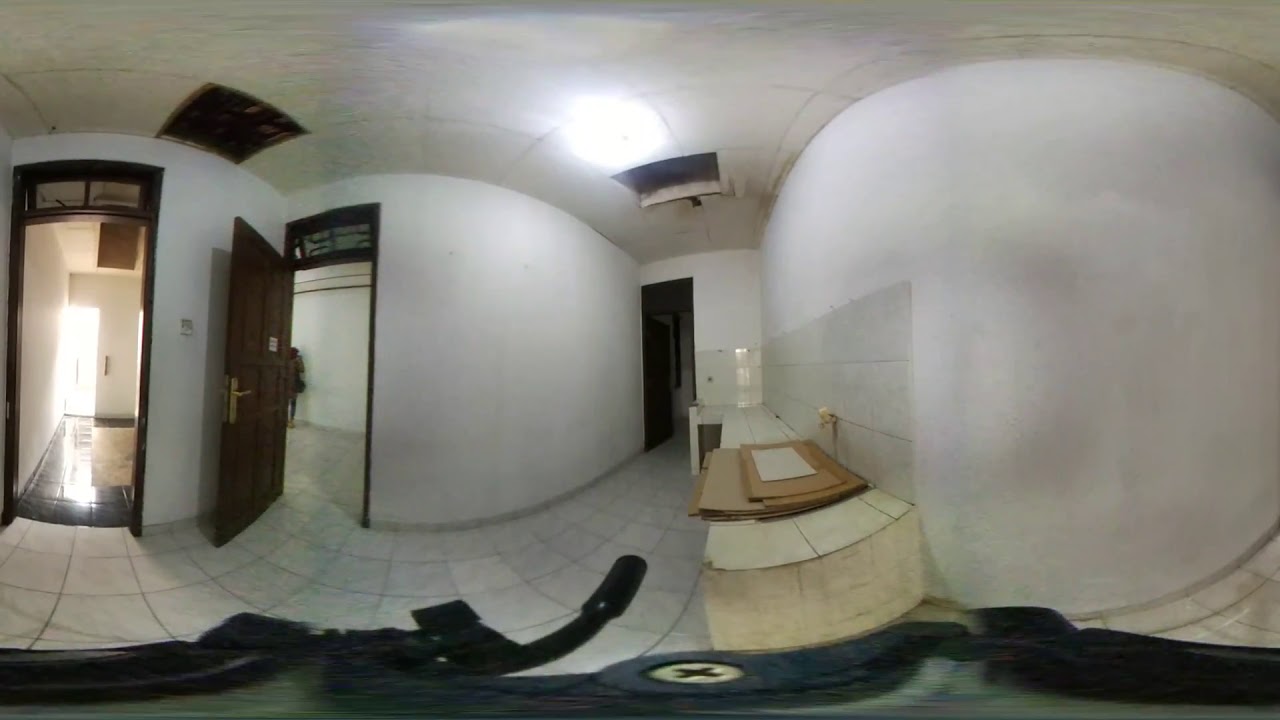The panoramic image depicts a minimally furnished room featuring all white walls, ceiling, and square white tile flooring. The warped perspective suggests it was captured with a 360-degree camera, possibly triggering a rounded curvature effect. On the left side of the photo, there's an open doorway emitting a bright, sunlit glow, hinting at an outdoor area or a well-lit adjoining space. Next to this door, another door with a large lever handle, similar to those in hotels, opens into a white wall. At the center of the image, an additional open doorway is framed in dark brown wood, consistent with the other door frames in the room. The middle of the photo reveals a large flat surface, resembling a kitchen table or counter, topped with a stack of cardboard. Included in the lower-left corner of the image are the edges of photography or motorbike equipment, such as handlebars and a gold screw head, indicative of the method used to capture the photograph. Noticeably, there are missing ceiling tiles on the left and center segments of the ceiling, adding to the room's somewhat incomplete appearance.